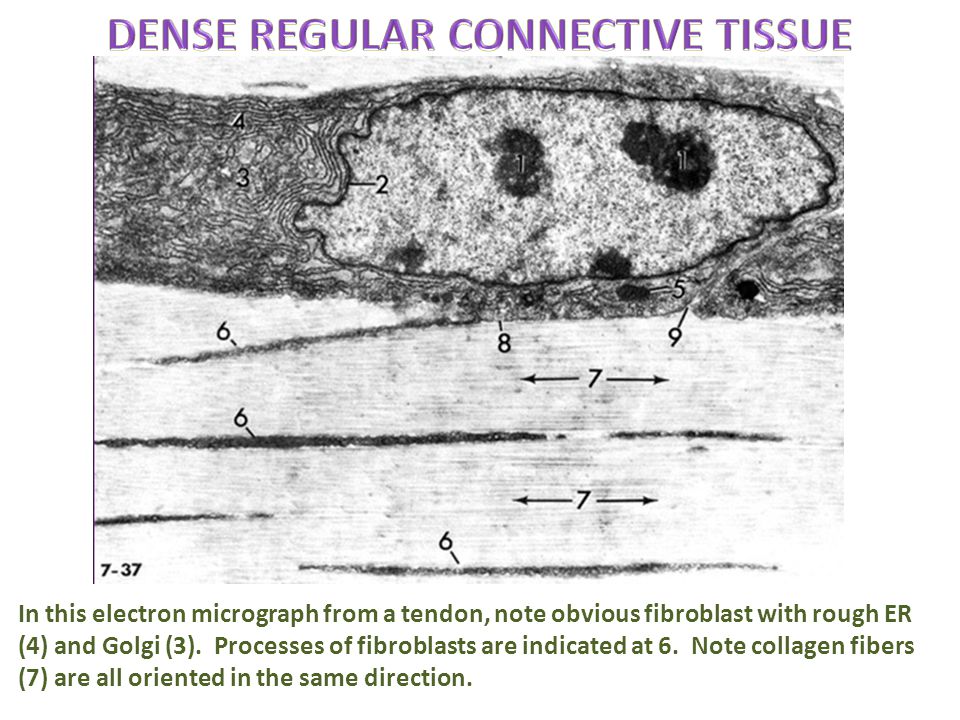The image is a detailed, scientific black and white slide that depicts a section of dense regular connective tissue. Prominently featured at the top in large, capitalized purple letters is the title "Dense Regular Connective Tissue." Below the heading, there is a rough, black-and-white illustration showing an elongated, rectangular tissue section with a large, irregular oval shape in the center, containing four black spots of varying sizes. Several arrows point to specific features of the tissue, marked with numbers. 

The bottom of the image includes a paragraph in green text that reads: "In this electron micrograph from a tendon, note obvious fibroblasts with rough ER (4) and Golgi (3). Processes of fibroblasts are indicated at (6). Note collagen fibers (7) that are all oriented in the same direction." This detailed description indicates a highly organized scientific infographic, showcasing various cellular components and their orientation within the tissue.